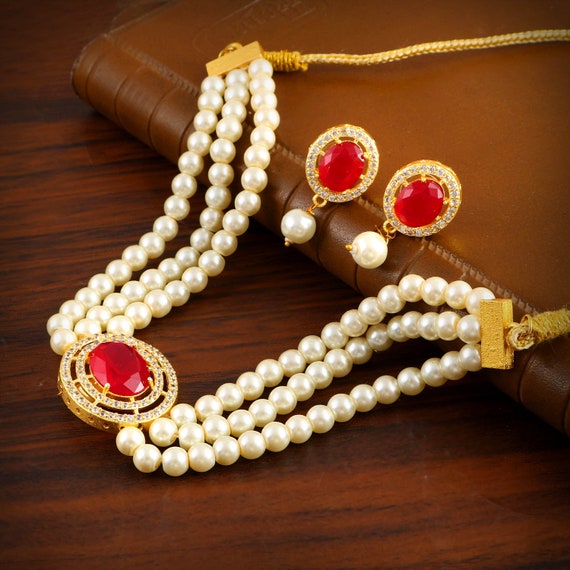This photograph showcases an exquisite jewelry set laid out on a dark wooden table, partially resting atop a leather-bound book. The centerpiece of the set is a stunning pearl choker necklace. This intricate piece features three strands of medium-sized, round, white pearls on each side, converging at a round central pendant. The pendant is beautifully crafted with two concentric circles of pavé-style diamonds, and at its center lies a striking red ruby, secured by delicate prongs. Flanking the pendant, the strands of pearls are anchored by two small gold blocks before transitioning into a gold cord, suggesting a tie-around neck design.

Accompanying the necklace are matching earrings, also showcased on the leather book. Each earring mirrors the necklace’s pendant, featuring a round ruby surrounded by pavé diamonds set in gold. Dangling gracefully from each earring is a single, lustrous white pearl. The meticulous craftsmanship and elegant design details, such as the visible prongs and gold settings, underscore the luxurious nature of this set.